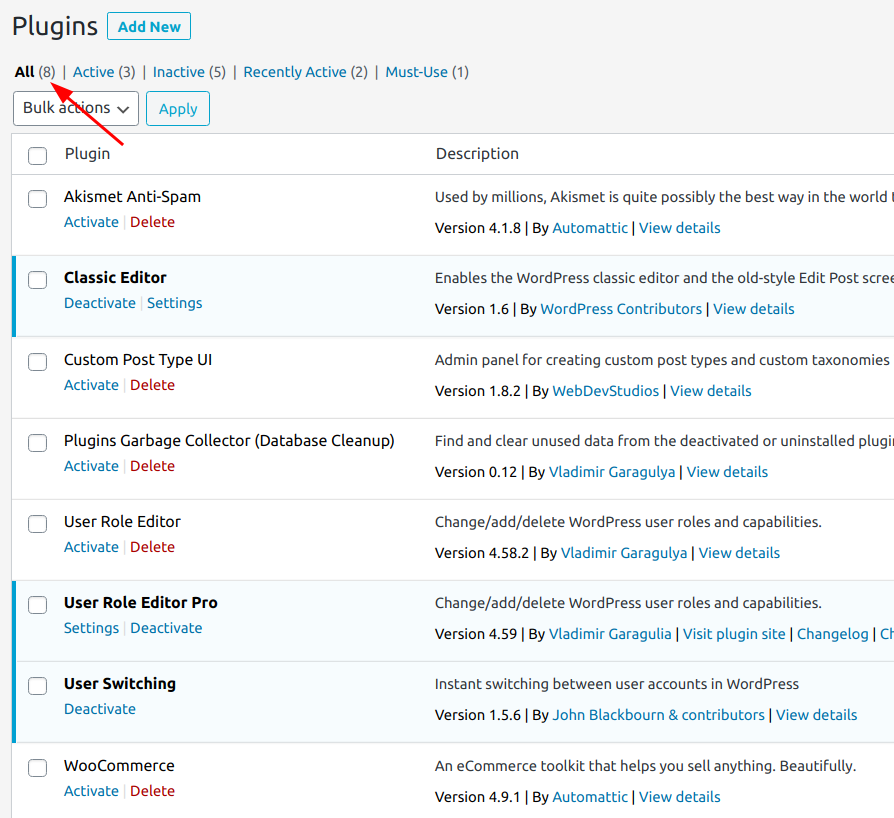The image depicts a user interface section for managing plugins. In the top left corner, there's the header "Plugins" in basic black text. To its right, a rectangular button with a blue outline and bold blue lettering reads "Add New."

Beneath this header, a series of menu options are listed horizontally, starting with "All" in bold black text, followed by a gray parenthetical number (8). This is separated by a gray line divider. Next, the word "Active" is in blue, indicating it's clickable, and has a parenthesis with the number (3), followed by another gray line divider. Continuing, the menu reads "Inactive" (5), "Recently Active" (2), and "Must-Use" (1), each delineated with gray dividers.

A red arrow is pointing upward from the section header labeled "Plugin" in bold, directing attention to the "All" option. Under the "All" option, a white rectangle with a black border contains the text "Bulk Actions" and a downward arrow, indicating a dropdown menu. To the right, a smaller rectangle with a light gray background and a blue border displays the word "Apply."

In the plugin section, a listing for "AKISMET Anti-Spam" appears in bold black text. To the left of this text is an unchecked tick box. Beneath "AKISMET Anti-Spam," the word "Activate" appears in blue, followed by a divider, and the word "Delete" appears in dark red on the far right. The plugin description below states, "Used by millions, AKISMET is quite possibly the best way in the world…" and is cut off. At the bottom of this section, "Version 4.1.8" is highlighted in bold text.